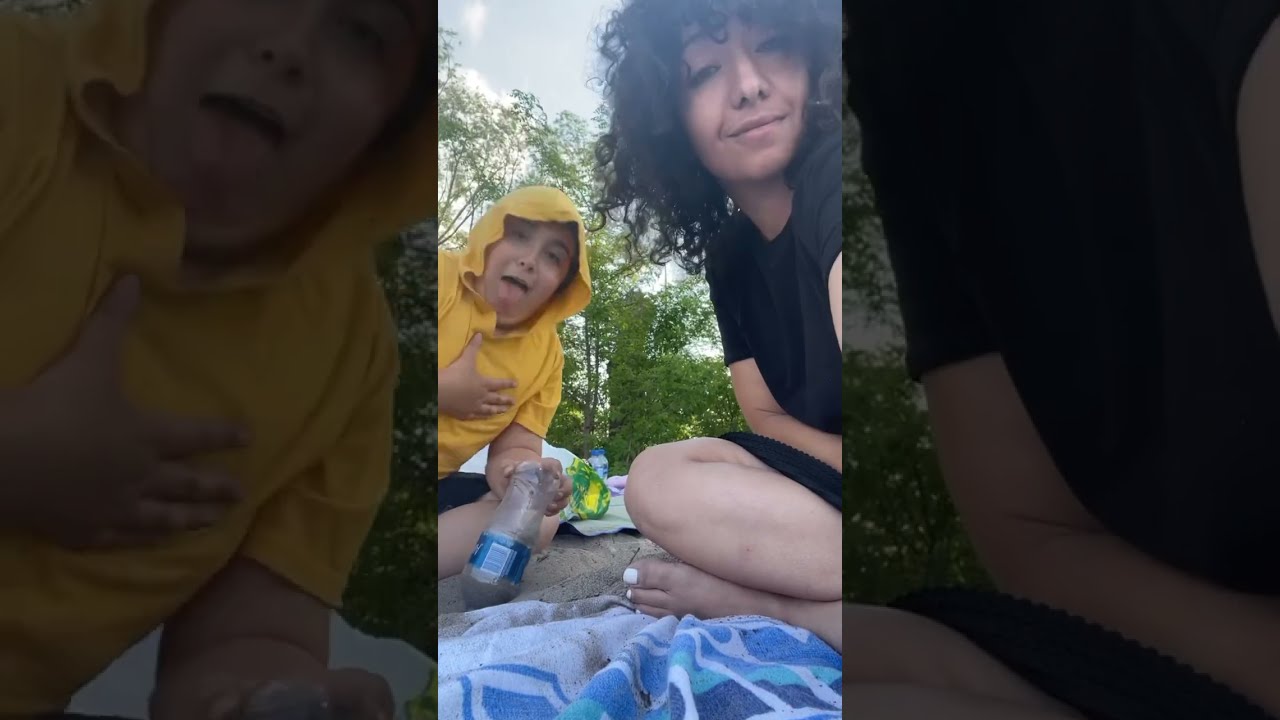The vertical cell phone image features two individuals seated in a sandy area, possibly a beach, with a backdrop of lush green vegetation and a partly cloudy sky. The person on the right is a woman with shoulder-length black curly hair and brown eyes, wearing a black shirt. She has a smirk on her face and sits cross-legged, emphasizing her blue painted toenails. To her left is a child in a yellow hoodie and short-sleeve shirt, also seated cross-legged. The child has brown eyes and is making a playful expression with his tongue sticking out. One of his hands rests on his chest while the other grasps a bottle filled with sand, which is placed on the ground. The image is framed by zoomed-in and tinted columns on either side: one highlighting the child's hand on his chest and the other focusing on the woman's elbow in contact with her black shirt. A partially sandy beach towel with white, blue, and teal colors lies at the bottom of the photo. Overall, the photograph is well-lit, depicting a sunny day with some clouds in the sky.